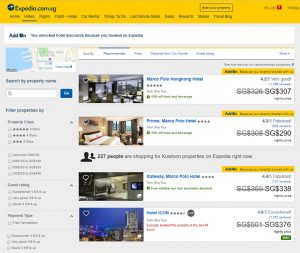Screenshot from Expedia.com.sg: 

This image is a detailed screenshot of a webpage from Expedia.com.sg, a website used for booking holiday accommodations and hotels. At the top of the page, there's a prominent yellow bar. The site's name, "Expedia.com.sg," is displayed in blue on the right, while the logo, a circular shape, is positioned on the top left side next to the word "Expedia." A narrow side panel on the left includes a small map at the top and a search bar underneath. Below this search bar, there are a series of filtering menus allowing users to select properties based on star ratings (three stars, four stars, or five stars). 

On the right side of the page, four hotel options are displayed as search results. In between the top two search results, a piece of information notes that "227 people are shopping for Kowloon," indicating popular demand. The search results pertain to hotels in the city of Hong Kong. Prices for these hotels are shown on the extreme right-hand side of the page in Singaporean dollars.